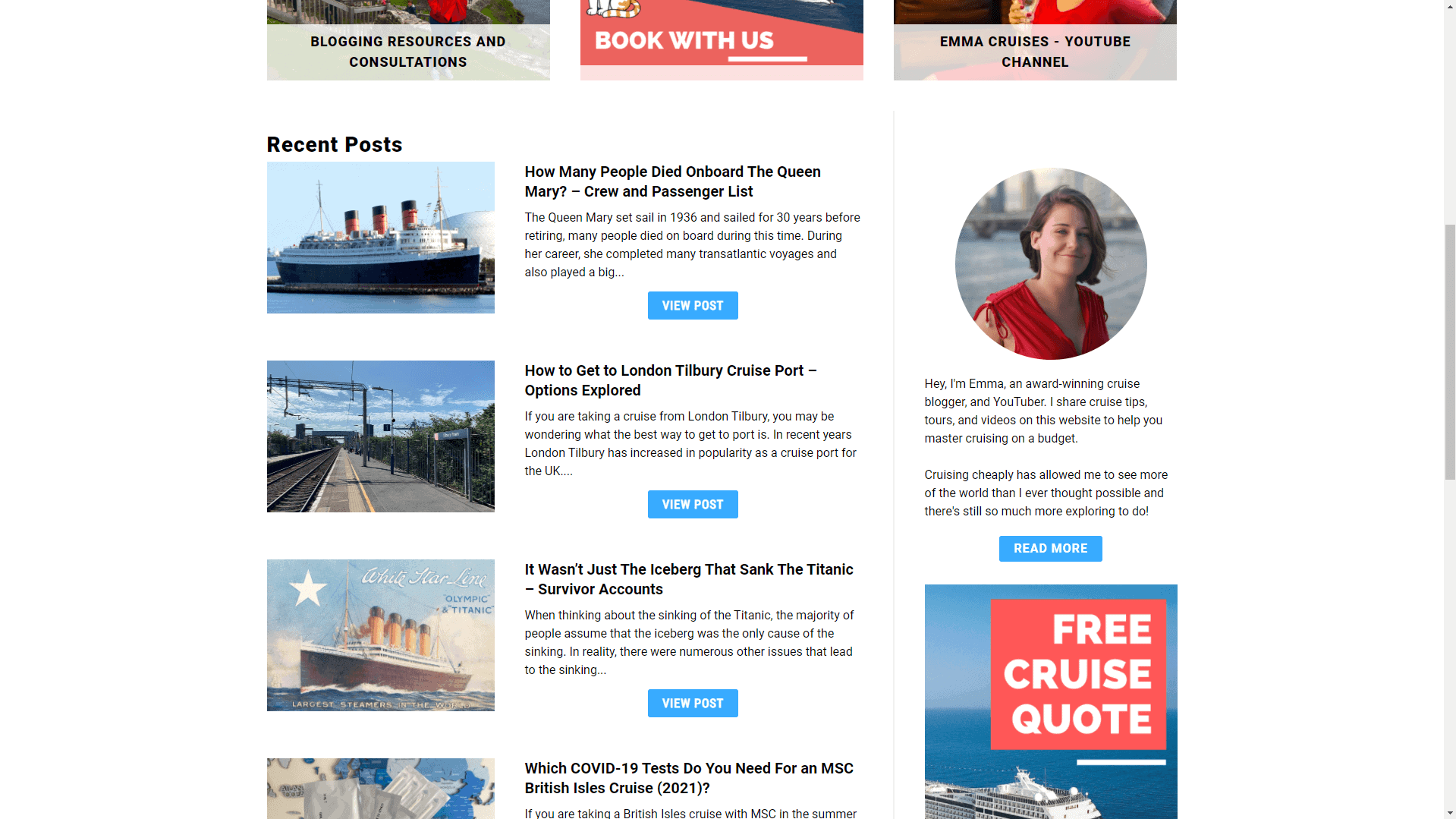This image is a cropped screenshot of a travel blog with a white background. At the top, the bottoms of three square images are visible, though their tops are cropped out. The leftmost box features the text "Blogging Resources and Consultations" in bold black font. The center box contains the text "Book with Us" in large white letters at its bottom left. The rightmost box reads "Emma Cruz's YouTube Channel" in bold black font.

Below these boxes, on the left side of the page, the section header "Recent Posts" is printed in bold black font. Under this heading, there is a vertical list of four blog articles. Each article includes a square thumbnail on the left, a title, an excerpt of the post, and a "View Post" button in blue on the right side of the excerpt.

To the right of the "Recent Posts" section, a thin horizontal gray line separates the blog articles from the blogger's bio. This bio section features a circular photo of the blogger at the top right, followed by a greeting message. At the bottom of the bio section, there is a center-aligned "Read More" link. Additionally, at the bottom right of the screenshot, the partially visible top of a box advertises a "Free Cruz Quote" in large white letters within a red background.